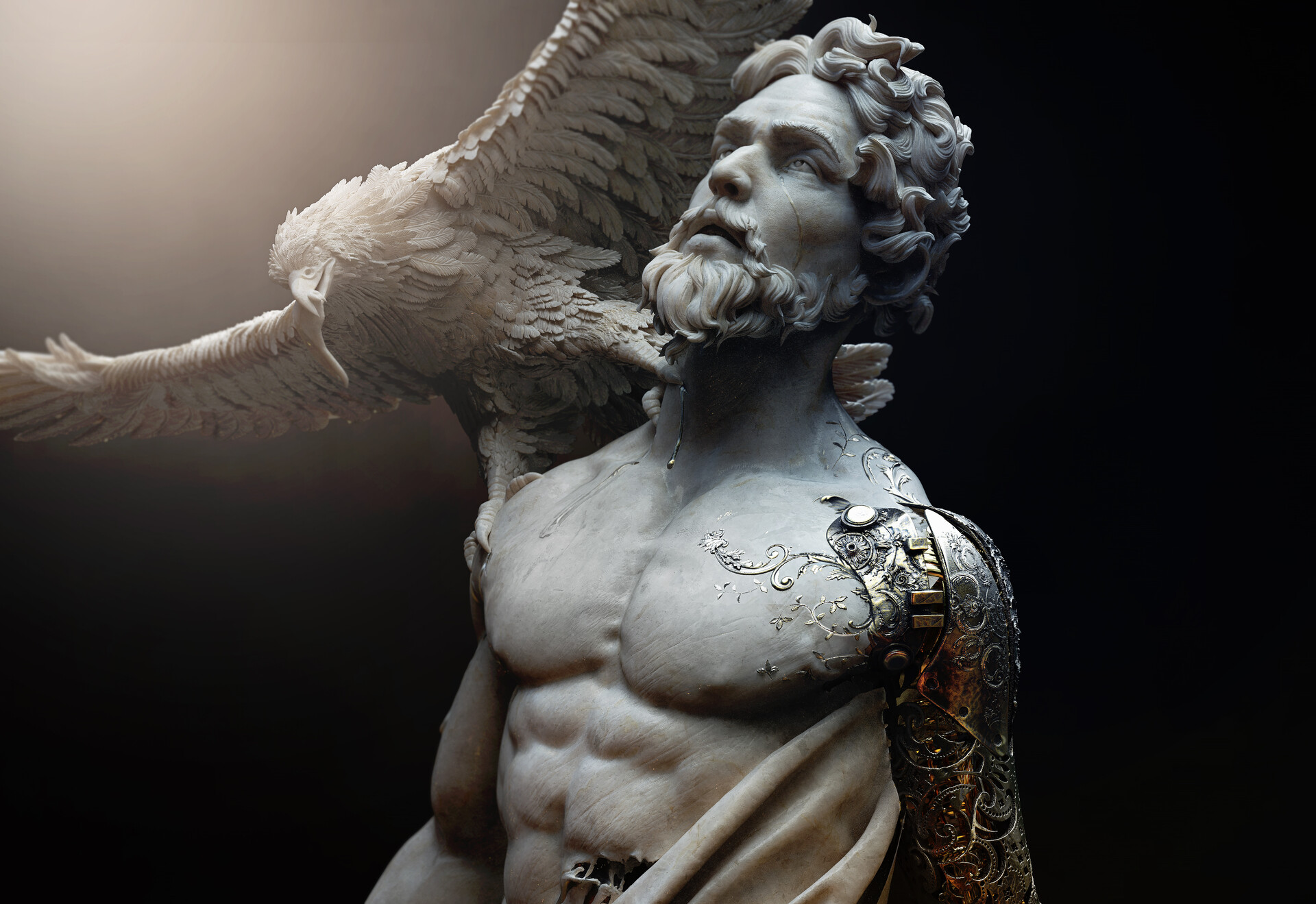The image features a highly detailed AI-generated sculpture of a man carved in a whitish-gray marble-like material. The man has short to medium-length curly hair and a thick curly beard and mustache. His left eye appears to be shedding a tear. The man's left arm is depicted as a mechanistic or cyborg-like limb, intricately composed of shiny gold gears, nuts, and bolts. He is shirtless, with a light cloth draped around the bottom half of his torso. Perched on his right shoulder is an eagle with its large wings spread wide, as if poised to take off or just landing. The artistry captures individual locks of hair and the feathers of the eagle, showcasing exquisite craftsmanship. The scene is illuminated by a light source from the upper left-hand corner, casting a subtle glow on the sculpture.